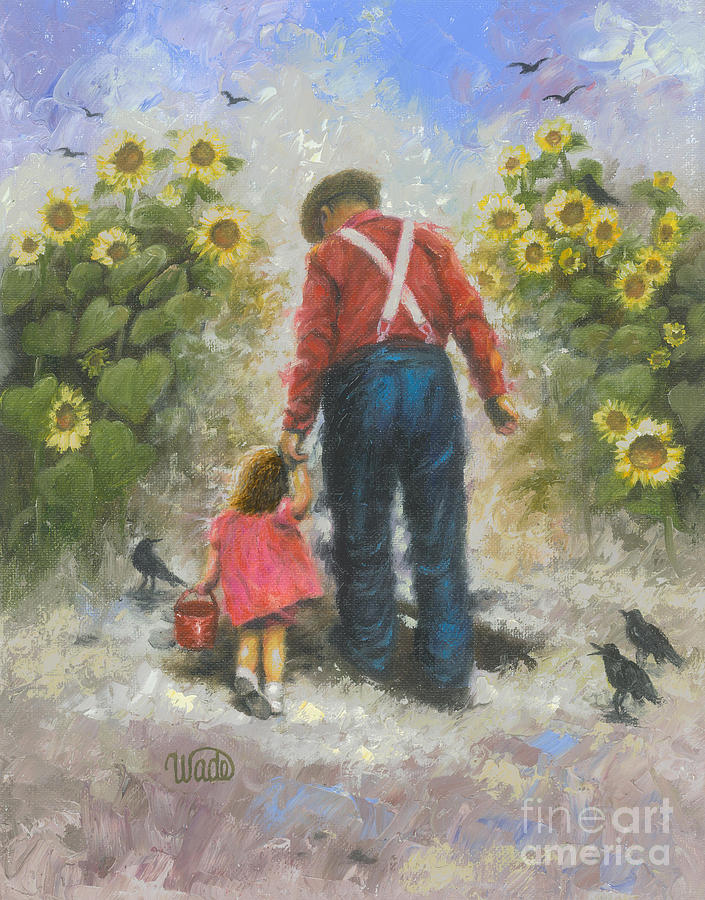This painting, titled by the signature "Wade" at the bottom left in green cursive, depicts a touching scene of a grandfather and his young granddaughter walking hand-in-hand through a field of towering sunflowers. The man, dressed in a long-sleeve red shirt with white suspenders cris-crossing his back over blue pants, gazes down lovingly at the little girl. He wears a hat, possibly a straw sun hat, shielding his face as they walk. The girl, dressed in a one-piece pink dress that reaches her bare knees, holds a red bucket in her left hand. Her delicate white socks and shoes stand out against the earthy ground beneath them. With her right arm outstretched, her hand is gently grasped by the man's left hand, guiding her through the scene.

The sunflowers surrounding them stretch above the man's head, their green stems and leaves framing the duo as they meander along the greyish-white path. In the clear blue sky with hints of purple and white, birds are spotted flying peacefully. On the ground, three black crows add a touch of activity, two positioned to the right of the man and one to the left of the girl. One crow appears animated, its beak open, possibly squawking at the pair. This artwork, part of the Fine Art America collection, captures a serene and heartwarming moment set against a natural canvas of towering sunflowers and a vibrant sky.